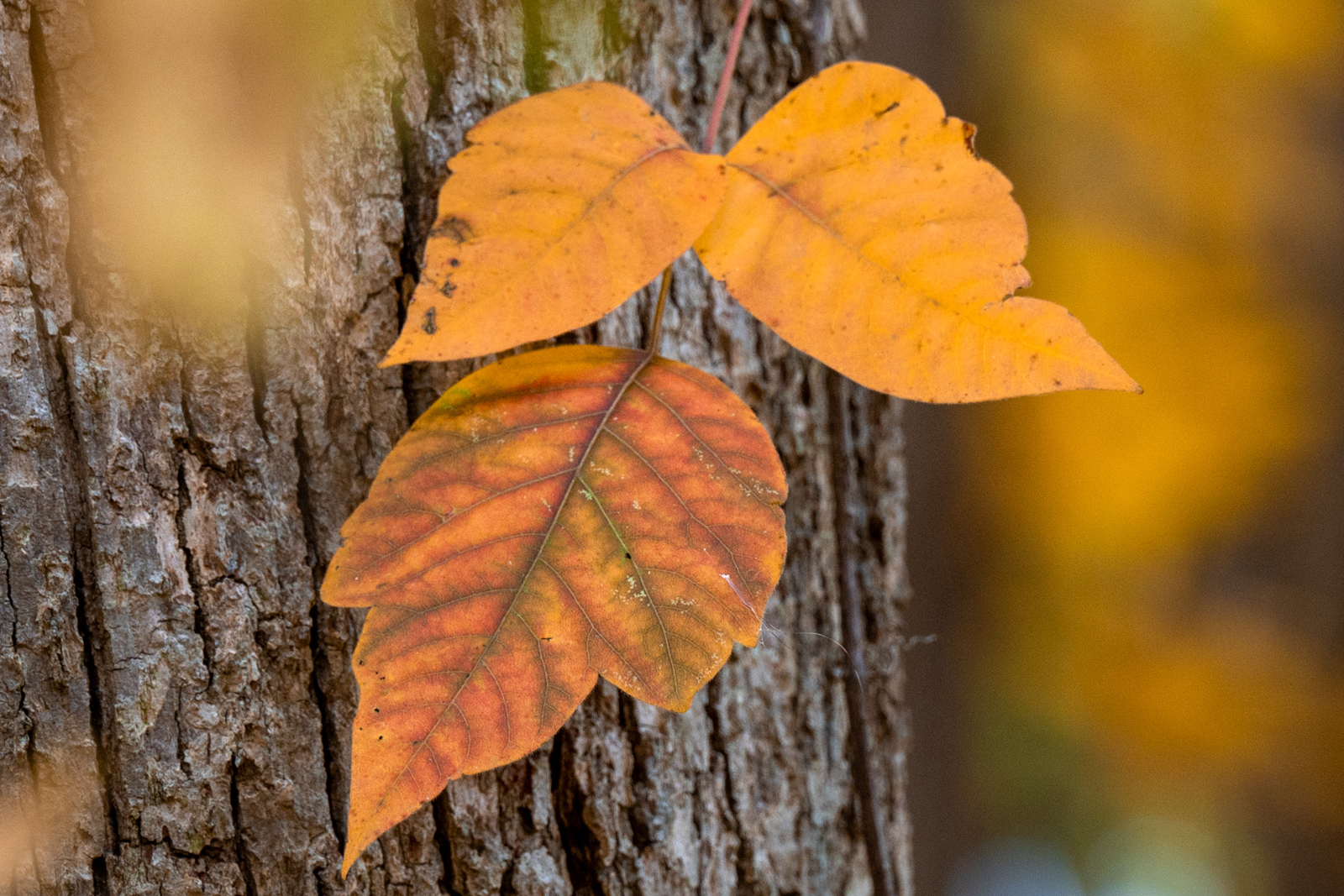This close-up image captures the essence of autumn with a detailed focus on the tree and its leaves. Dominating the center are three leaves; the top two leaves are a golden yellow with subtle serrations, displaying prominent dark veins with hints of green, while the bottom leaf features a blend of orange with traces of brown and green, showing a slightly more rounded shape. The leaves are sharply in focus against a backdrop of a tree trunk with thick, rugged bark in shades of brown and gray. The surrounding background, including other leaves and parts of the tree, is heavily blurred, rendering them into mere blobs of autumnal colors - oranges, reds, and yellows, which enhances the vividness of the central leaves. The blurred elements evoke a sense of depth and draw more attention to the intricate details of the focal leaves, encapsulating the vibrant fall foliage reminiscent of a serene autumn day.